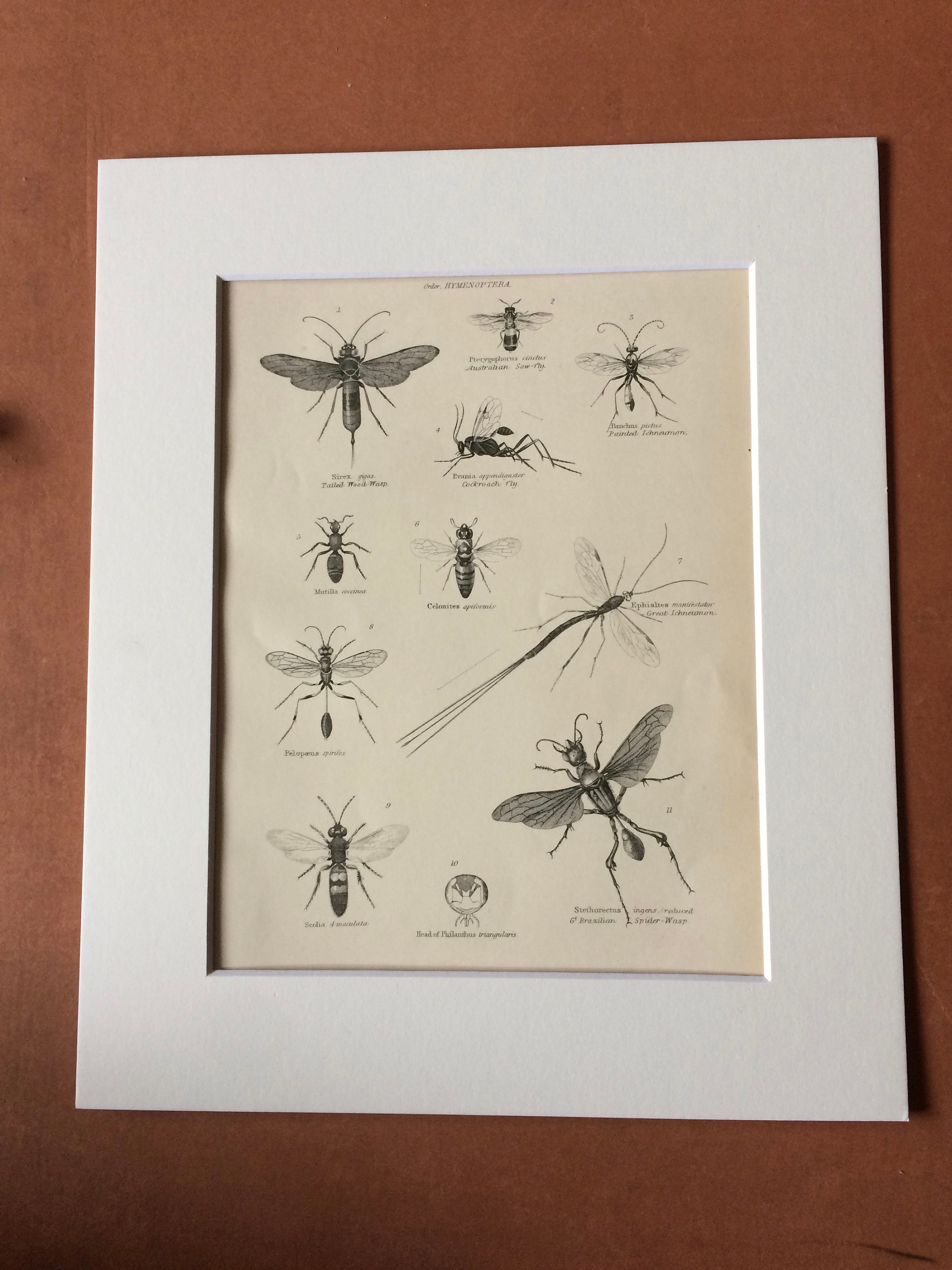In this detailed photograph, a white-framed display showcases an assortment of flying insects, meticulously arranged in rows. The frame encloses an impressive collection of 11 different species, each positioned with precision. Underneath each insect, tiny labels denote their names, though the text is too small to discern clearly in the image. The arrangement is centered on a wall painted in a rich, reddish-brown hue, providing a warm contrast to the crisp, white frame. The artwork is prominently placed, dominating the center of the photograph. This image appears to have been taken in someone's home, capturing the unique and detailed portrait of these fascinating flying insects.